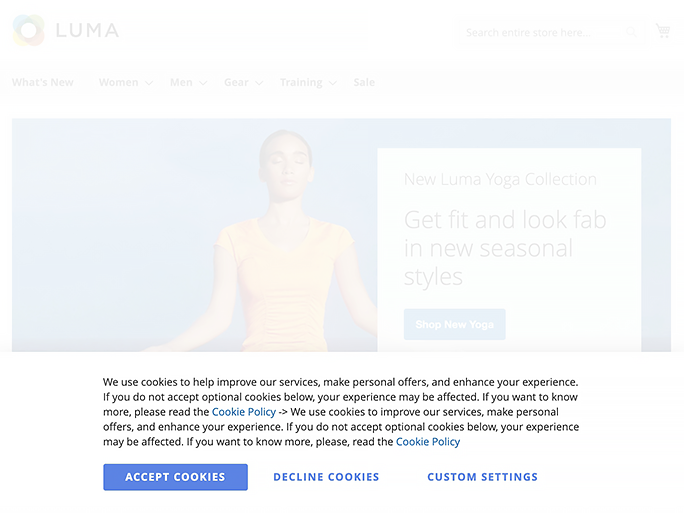Screenshot from a website caught under a white overlay, predominantly featuring a partially obscured image of a meditating woman. Positioned in the lotus pose with eyes closed and hands relaxed by her sides, her slicked-back hair is barely visible through the overlay. The top left hosts the Luma logo, accented by thin text and colored geometric shapes. Accompanying the visual is text on the right side that reads, "In the new season, get fit and look fab with new seasonal styles. Shop our new yoga gear." A noticeable banner at the bottom addresses cookies policy, providing options to 'Accept Cookies,' 'Decline Cookies,' and customize settings. It reads: "We use cookies to help improve our services, make personal offers, and enhance your experience. If you do not accept optional cookies, your experience may be affected. To learn more, please read our cookie policy," with the "cookie policy" being a clickable blue text link.